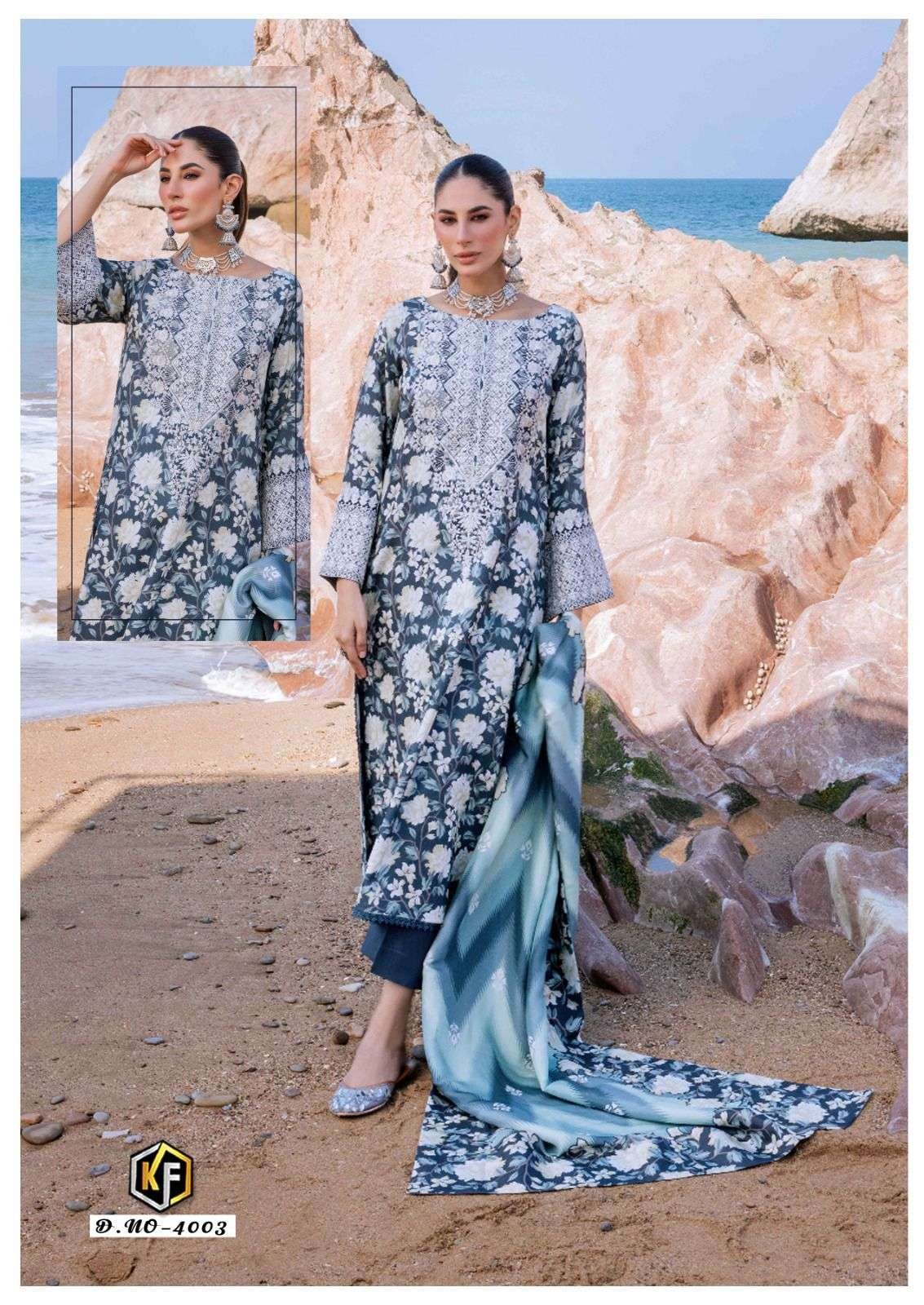In this advertisement for an elegant dress, a medium-aged woman with dark, slicked-back hair stands gracefully on a beach with dramatic tan rock formations and the blue ocean against a clear sky in the background. She wears a striking blue and white dress that features intricate floral patterns, reminiscent of Indian or Middle Eastern designs, with lace detailing at the cuffs and navy blue pants underneath. Her outfit includes matching blue flats and a silver choker paired with dangly silver and navy earrings. In her left hand, she holds a coordinating scarf. An inset at the top left corner displays a close-up of her torso, showing her holding her right hand to her forehead. The bottom left corner of the image includes text in gold and silver, reading "KF" and "D No/403".